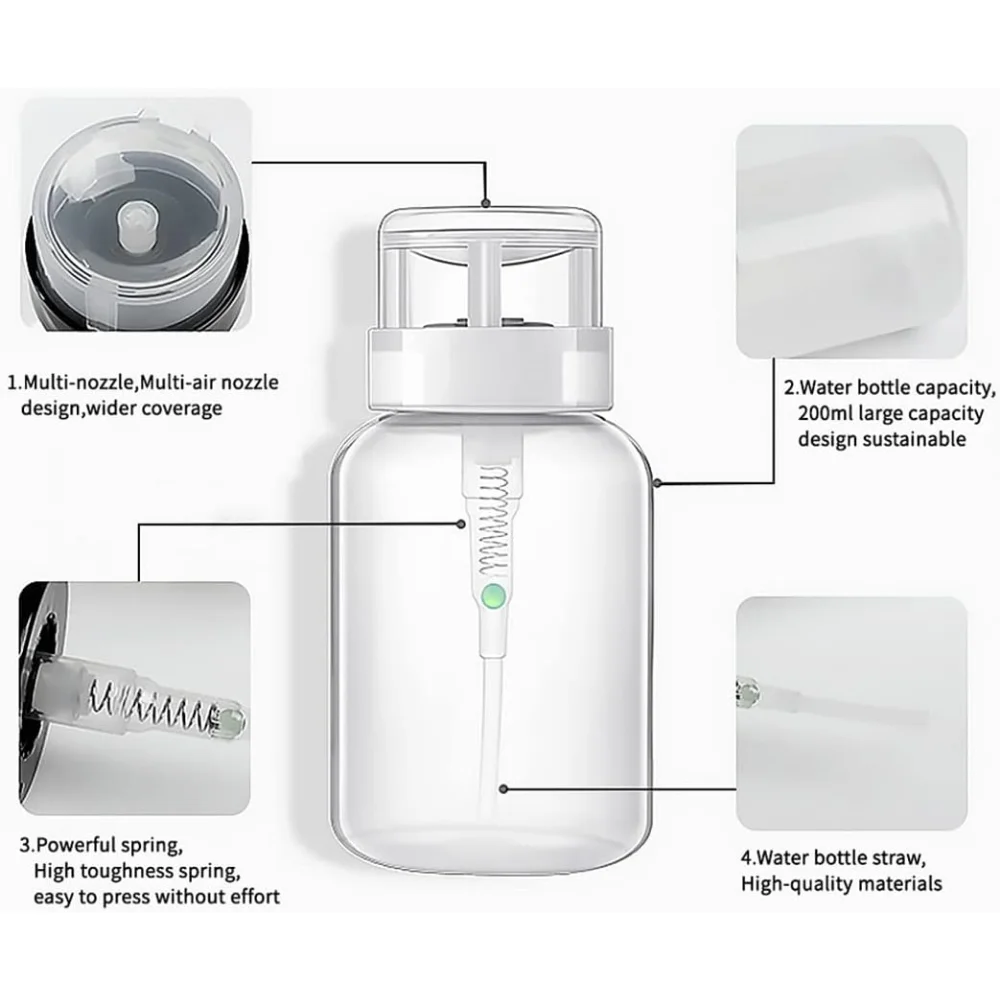The image showcases a transparent water bottle positioned centrally against a solid white background, without any border. The water bottle features a screw-style, see-through lid with a pump mechanism that includes a visible spring inside a plastic casing. Surrounding the main container are four smaller square images, one in each corner, each highlighting different features of the bottle. 

- The upper left square details the lid and is captioned "Number 1: Multi-nozzle, multi-air nozzle design, wider coverage," with an arrow pointing to the lid.
- The upper right square highlights the container's capacity, labeled "Number 2: Water bottle capacity, 200 ml, large capacity design, sustainable," with an arrow indicating the bottle.
- The lower left square focuses on a close-up view of the spring inside, described as "Number 3: Powerful spring, high toughness spring, easy to press without effort."
- The lower right square shows the spout and is captioned "Number 4: Water bottle straw, high quality materials," with an arrow pointing to the specific part.

The color palette of the image includes white, off-white, light gray, and black, creating a clean and modern informational design.